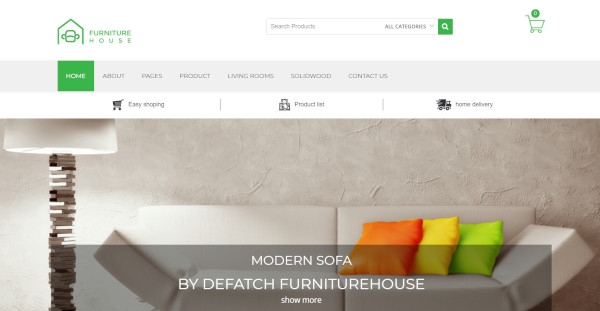The image showcases the homepage of a website called "Furniture House," characterized by a sleek and modern design dominated by white, green, and gray hues. In the upper left corner, the brand name "Furniture House" is prominently displayed alongside a minimalist green outline of a house logo. 

Central to the page is a stylish, modern-looking gray sofa situated in a room with a textured cement wall. The sofa has a distinctive "smile" shape, with its corners elegantly curved upward. Beside it stands a uniquely designed lamp that complements the contemporary aesthetic.

The website interface features a search bar centered on the page, currently set to search across all categories, with a conspicuous green 'Search' button adjacent to it. A cart icon, currently empty, is also visible. Beneath the search section is the main navigation menu, which includes links to Home, About, Pages, Products, Living Room, Solid Wood, and Contact Us sections. 

Additional information on the homepage highlights services like Easy Shipping (possibly "Etsy" Shipping), Product Lists, and Home Delivery options. A label on the sofa image reads "Modern Sofa by Defetch Furniture House," accompanied by a 'Show More' button for additional details.